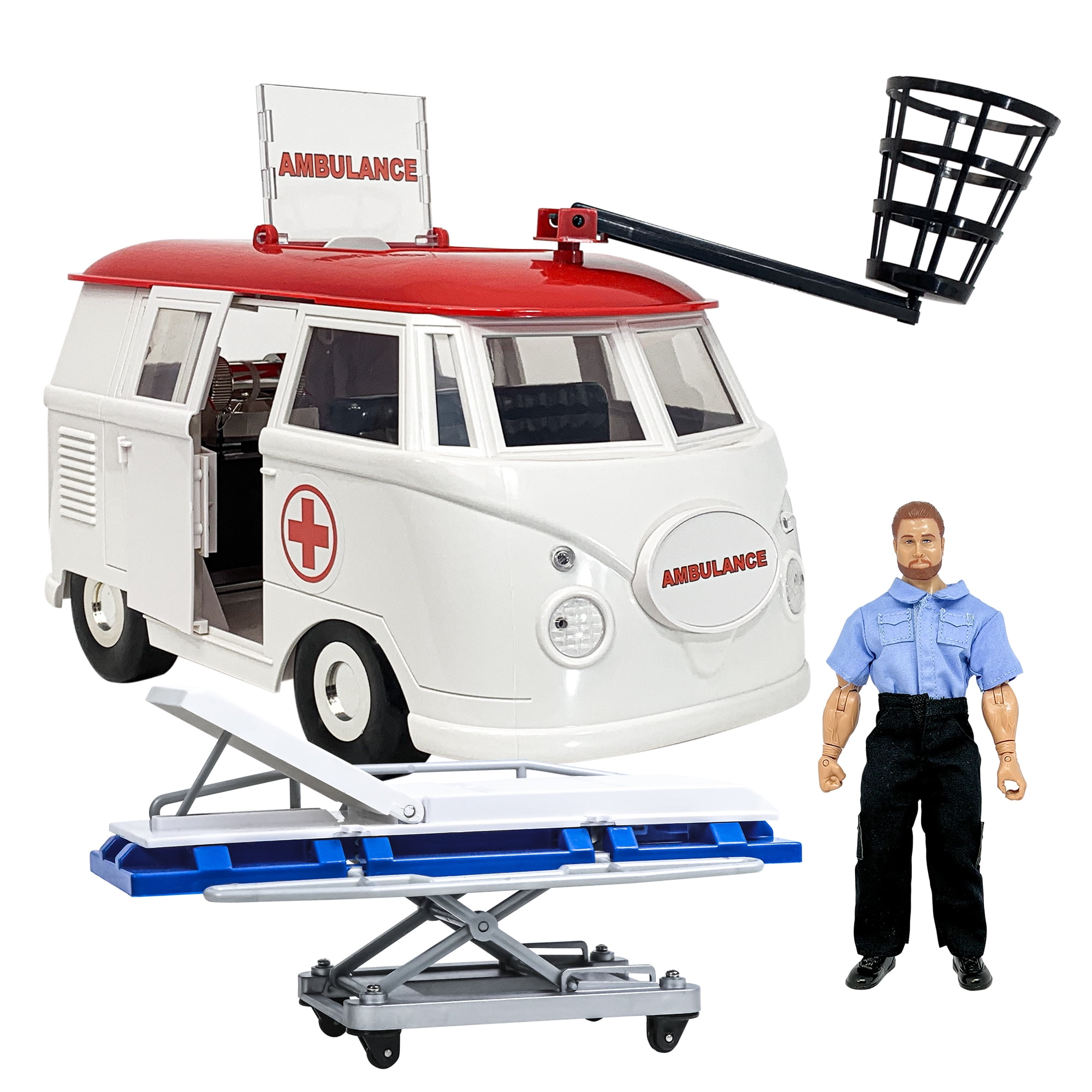The image showcases a toy ambulance modeled after a 1960s Volkswagen bus, repurposed with several detailed features. The ambulance, with a striking red roof and clear plastic signage that says "Ambulance" on the front, also bears the word "Ambulance" on the front grill and a red cross enclosed in a circle on the left side. An open side door reveals the toy's interior. Affixed to the top of the ambulance is a black steel-like basket mounted on a crane-like arm, although the setup appears somewhat impractical. At the base of the ambulance, there is a gurney made of painted metal and plastic, featuring blue, white, and grey colors with black wheels. To the right of the gurney stands an action figure clearly designed to be one of the ambulance rescuers. This figure is dressed in a collared, short-sleeved blue shirt paired with black slacks and shiny black boots. The figure sports a handlebar mustache that merges into a beard and has short brown hair. The detailing even extends to the toy's articulated arms, allowing for movement at the joints.